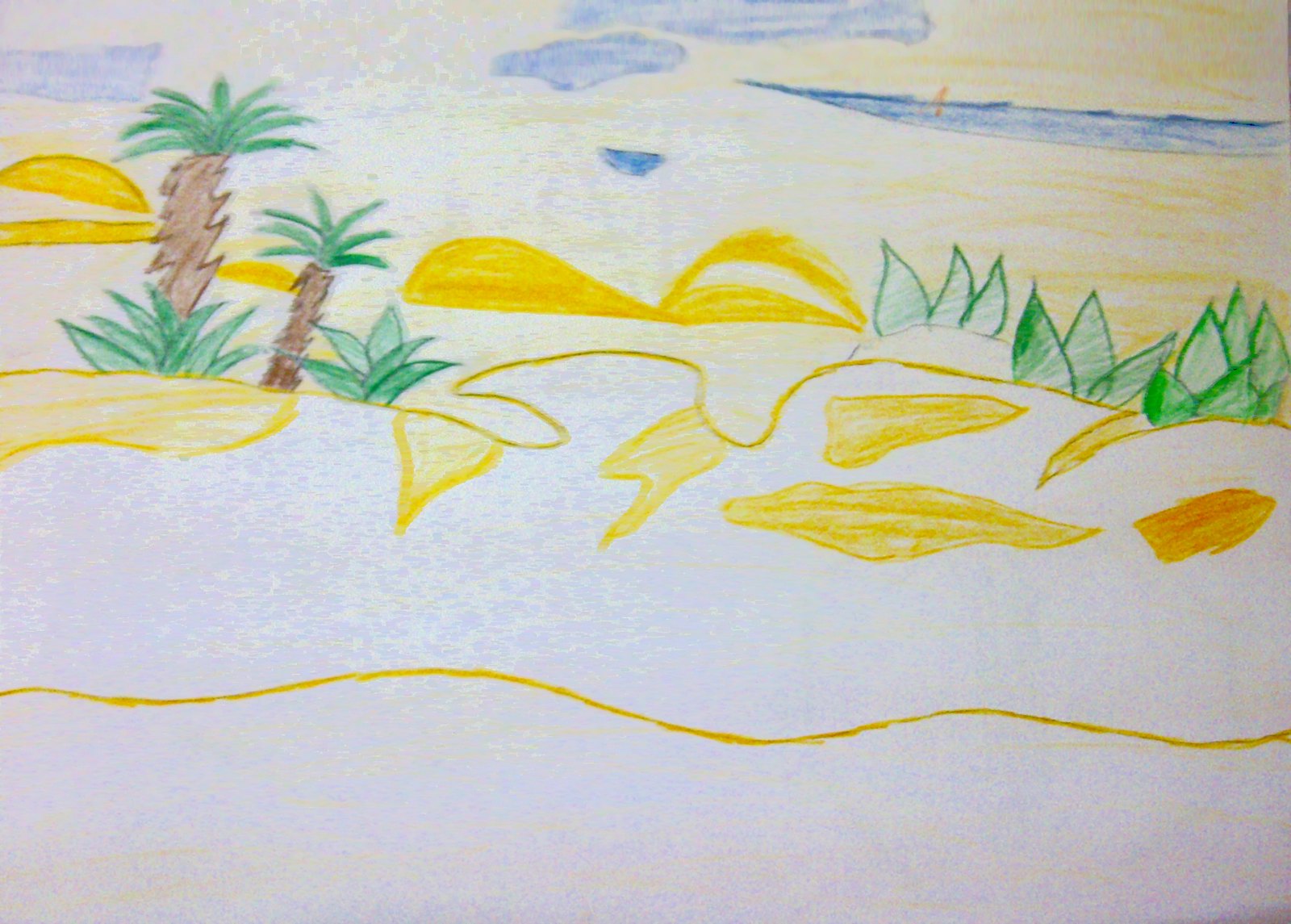This vibrant drawing, created by a child using yellow, red, blue, brown, and green colored pencils, depicts a picturesque scene of the Sahara Desert. The bottom portion of the artwork features light yellow shading, suggesting a sandy terrain. Prominently drawn in the center with brown pencil is a large palm tree, its crown adorned with lush green leaves. At the base of the palm tree, additional green foliage is visible, enhancing the desert oasis feel. The background showcases small blue peaks and scattered blue areas, representing the presence of distant water bodies or ocean waves, adding depth and contrast to the scene. The thoughtful use of color and detail highlights the child's imaginative and expressive interpretation of a desert landscape.